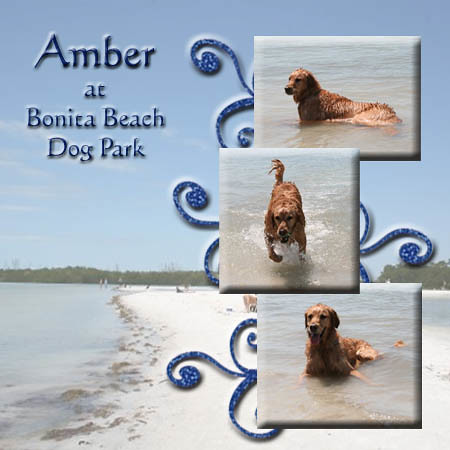This image is a commemorative montage titled "Amber at Bonita Beach Dog Park," prominently displayed in dark blue text in the upper left corner. The right side of the image features three staggered photographs of Amber, a golden retriever, enjoying the beach. In the top image, Amber faces left while standing in water that reaches halfway up her body. The middle image captures her running straight towards the camera through the water, and the bottom image shows her lying down in the water, facing forward. The background beneath these pictures reveals a vivid beach scene with lush greenery at the back, pristine white sand, and inviting, clear blue water. The photos are laid over a subtle, blue, squirrel-like design that complements the overall beachy aesthetic.